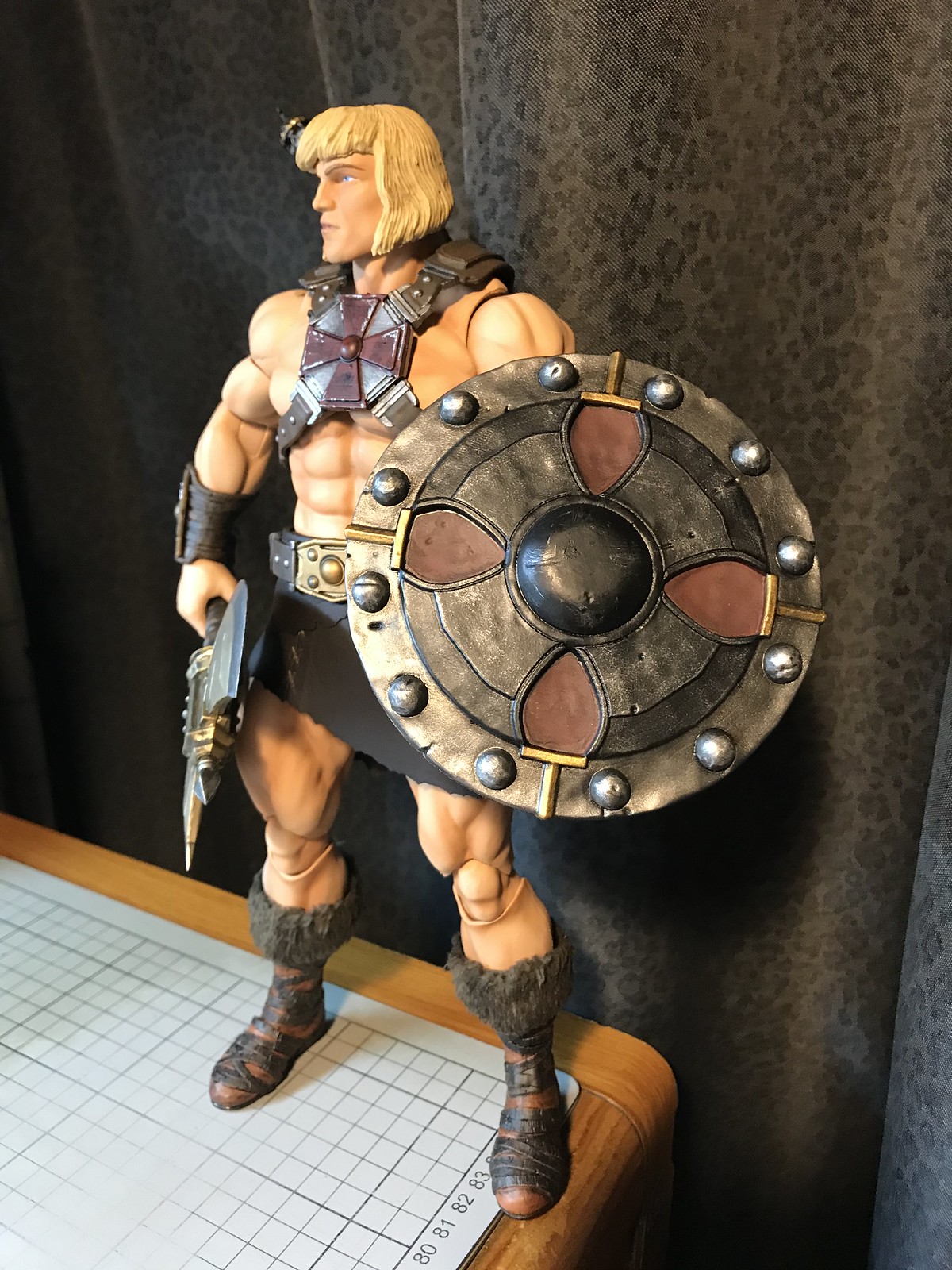This indoor photo features a highly detailed action figure of He-Man from the television series "He-Man and the Masters of the Universe." Centered in the image, He-Man stands against a dark, cheetah-print curtain, positioned on a wooden table that has a mat with numbering (80, 81, 82, 83) and a lined graph pattern across it. The He-Man figure boasts pronounced muscular definition and is shirtless, showcasing his iconic muscular build and blonde hair that extends to his jawline, with some strands slightly out of place.

In his left hand, He-Man wields a large, ornate shield adorned with rivets arranged in a cross pattern, while his right hand grips a detailed, two-bladed battle axe. His attire includes a brown breastplate featuring another cross insignia, a belt, and a short skirt-like garment. His boots are intricately designed, featuring crisscross leather straps and furry tops, along with visible rust marks and other intricate detailing on his equipment. The photograph appears to be taken to display or potentially sell this meticulously crafted figure, emphasizing its elaborate design and craftsmanship.